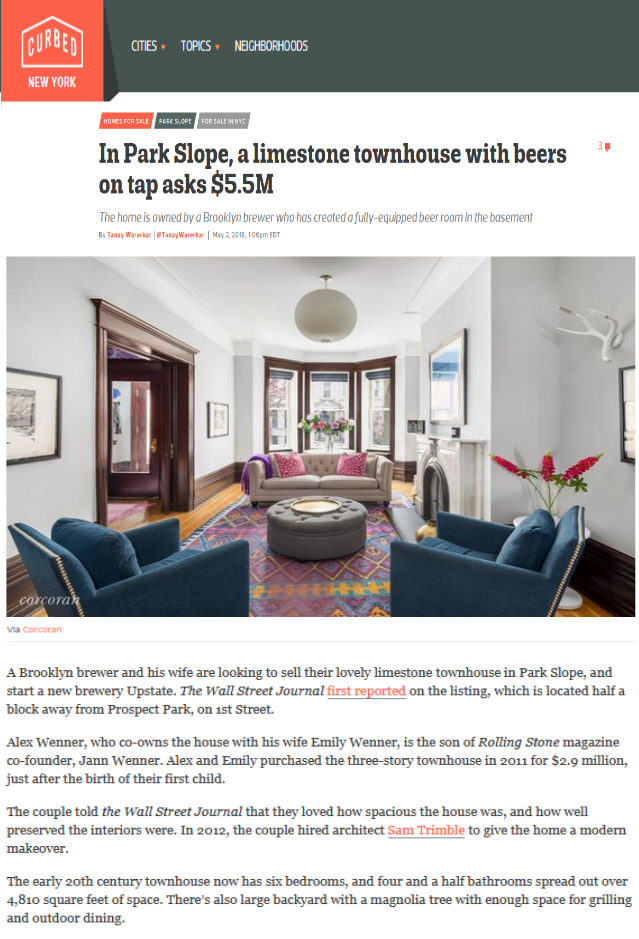Captured against a pristine white background, the focal point is an orange square highlighting the words "New York," "Curbed," and "In Park Slope." This detailed description chronicles the sale of a limestone townhouse in the Park Slope neighborhood of Brooklyn. The property, listed at $5.5 million, features a tastefully decorated living room with two chairs and a couch. The listing is prominently covered by The Wall Street Journal, emphasizing its prime location just half a block from Prospect Park on First Street.

The townhouse belongs to Alex and Emily Weiner. Alex is a notable figure, being the son of Rolling Stone magazine co-founder Jan Weiner. The couple acquired the three-story limestone home in 2011 for $2.9 million. Alex, a Brooklyn brewer by profession, and his wife Emily are selling the property to pursue their dream of opening a new brewery upstate.

The scene encapsulates a blend of historic charm and modern entrepreneurial spirit, indicative of the evolving Brooklyn neighborhood.